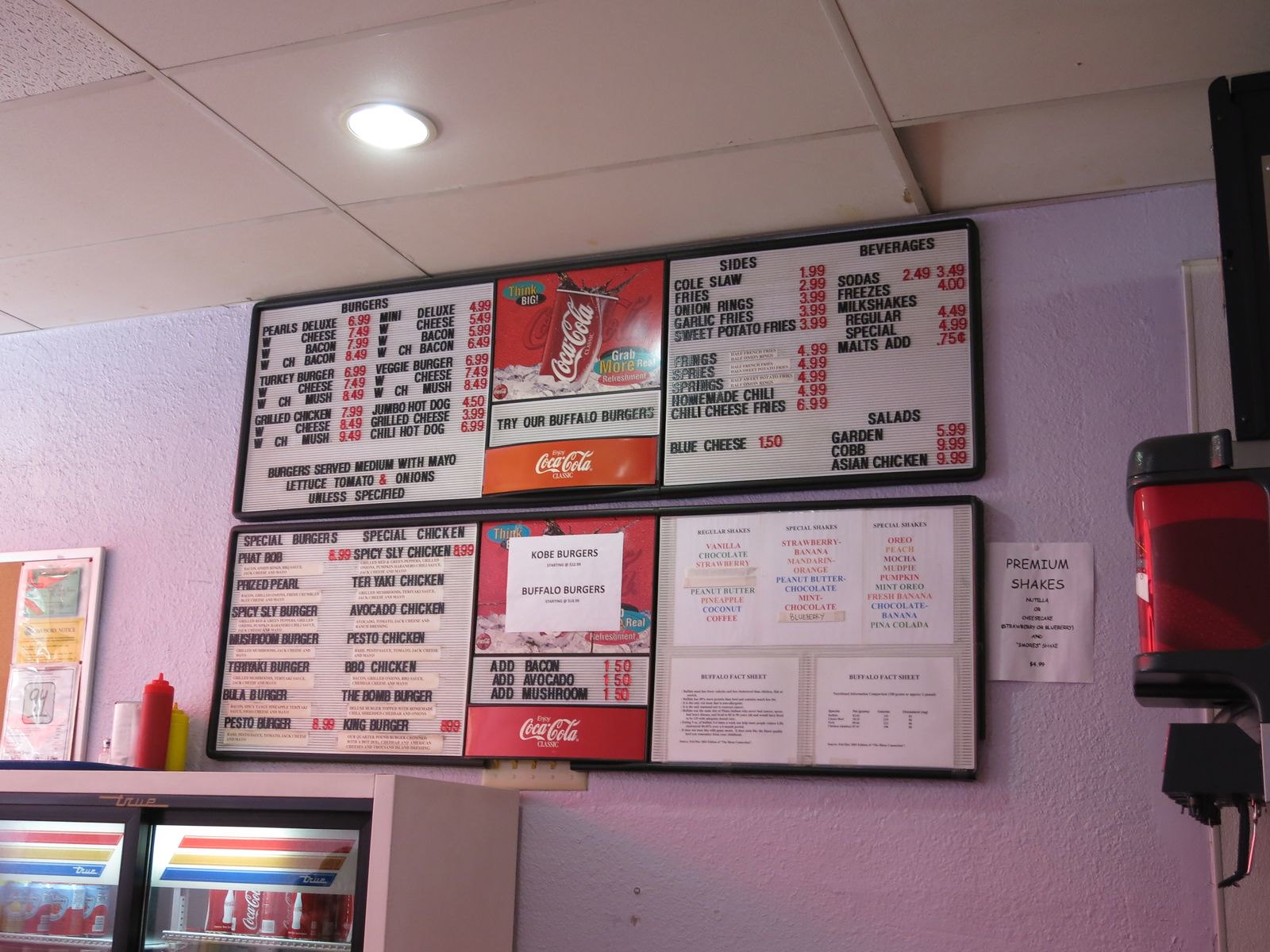The image depicts an interior view of a casual dining establishment, likely a diner or café. The setting features a white, textured wall and a ceiling composed of white or off-white tiles. Some of the ceiling tiles are slightly displaced, and one includes recessed lighting.

Mounted on the wall are two menu boards with manually placed black letters. The top menu board prominently advertises items such as deluxe cheeseburgers, bacon burgers, turkey burgers, grilled chicken sandwiches, jumbo hot dogs, grilled cheese sandwiches, and chili hot dogs. The description specifies that all these items are served with mayonnaise, lettuce, tomato, and onions unless stated otherwise. The prices on the menu are highlighted in red.

In between the two menu boards, there is a Coca-Cola advertisement promoting buffalo burgers. The lower menu board lists daily specials, including teriyaki chicken and pesto chicken. Additionally, there are several printed paper signs affixed to the wall, though their contents are not clearly legible.

In the foreground, there is a refrigerated display cabinet containing various beverages, including cans of soda. To the right of this setup, part of a soda dispensing machine is visible, completing the functional dining space designed to offer quick and varied meal options.